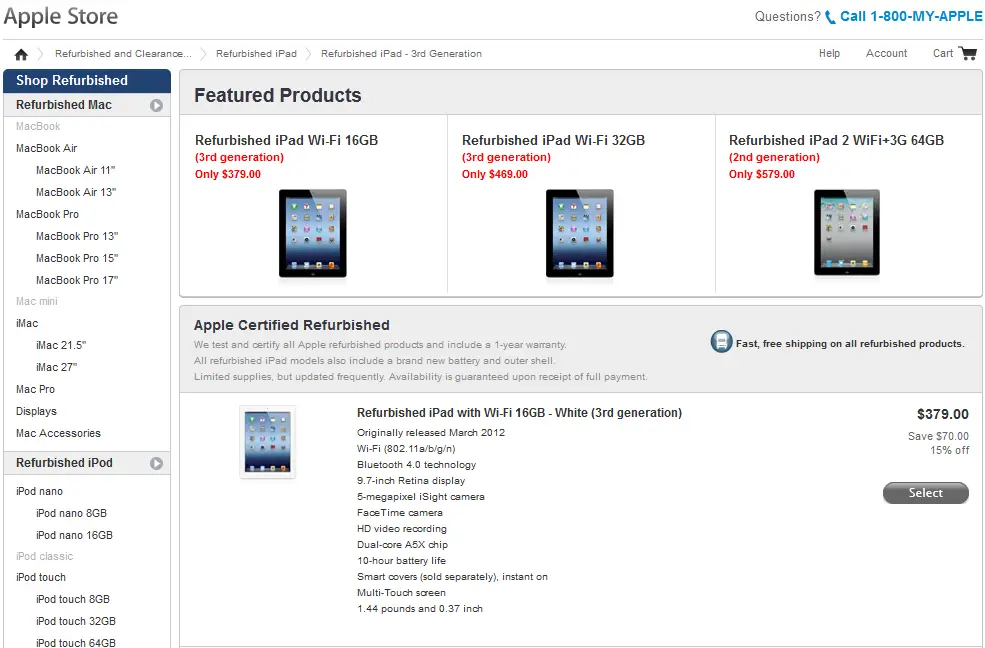A screenshot of an Apple Store online interface is neatly presented. At the top left corner, "Apple" is displayed in gray, with a contrasting white banner to the right, featuring questions written in gray. Adjacent to this is an icon of a phone, along with the helpline number "1-800-MY-APPLE" in blue. Below this banner are various navigation buttons in gray, including "Home," "Refurbished and Clearance," "Refurbished iPad," "Refurbished iPad 3rd Generation," showcasing a user's recent search activity. Other buttons include "Help," "Account," and "Cart."

The left side of the screen offers a shop-by-category menu, listing options such as "MacBook Airs" in 11 and 13-inch sizes, "MacBook Pros" in 13, 15, and 17-inch sizes, "Mac" in 21.5-inch and 27-inch sizes, "Mac Pro Displays," "Mac Accessories," and "Refurbished iPods." Centered prominently are specific results for "Refurbished iPad 3rd Generation," displaying three different options: a 16GB model for $378, a 32GB model for $488, and a 64GB model for $679. The user has evidently shown interest in the $379 16GB model, clicking it for more information, with an option to select and proceed with the purchase.